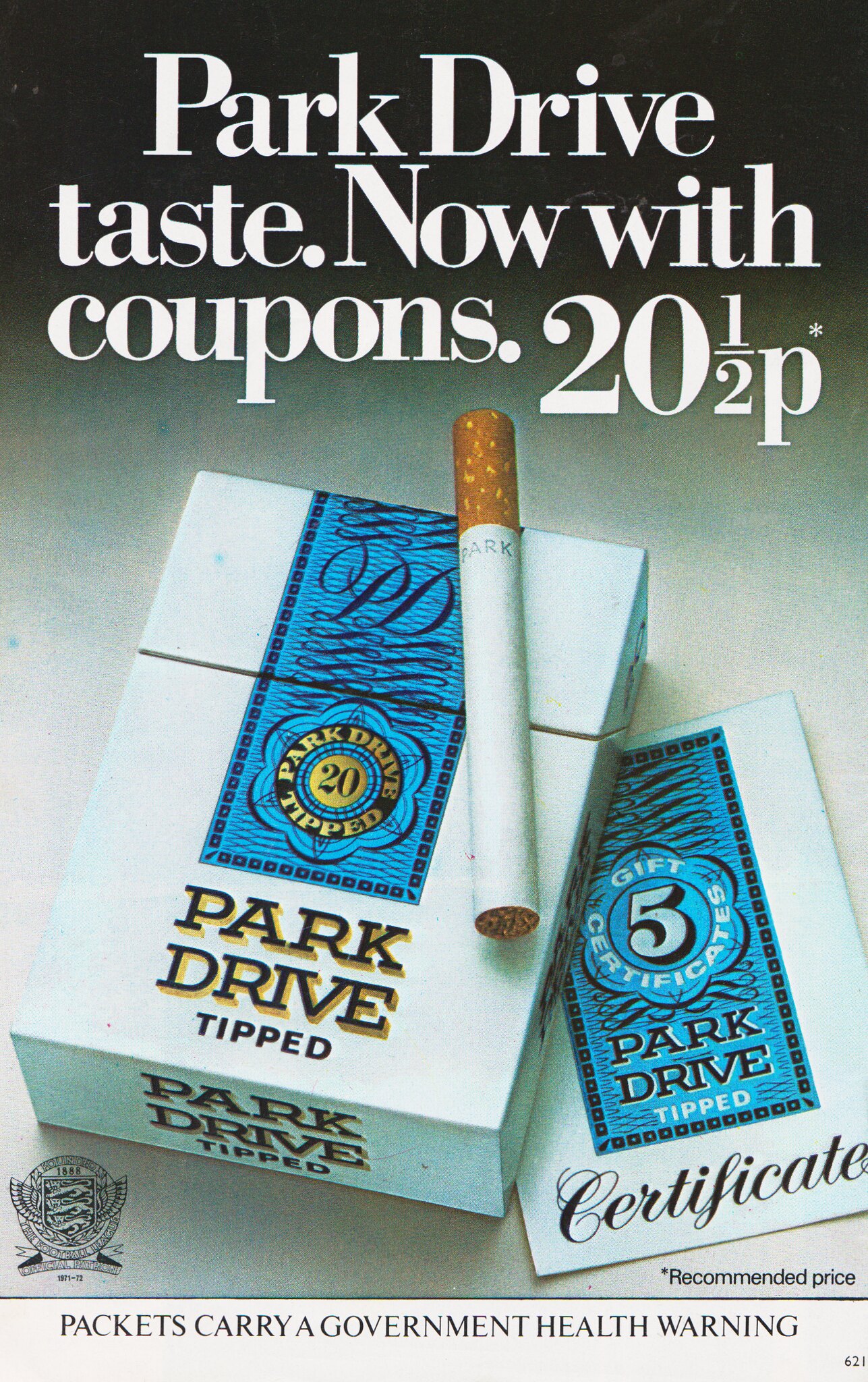The image depicts an advertisement for Park Drive tipped cigarettes, likely from the late 1970s to early 1980s. The focal point is a white box of Park Drive cigarettes, adorned with a prominent blue sticker that extends from the top down to the box itself. The sticker features an elaborate design with swirls and boxed patterns, and prominently displays "PD" for Park Drive. Below this, encased in a black circle with gold lettering, it reads "Park Drive tipped." The central portion of the design states "20 gold," with the text "Park Drive tastes now with coupons 20 1/2 P" prominently featured.

To the right, there is a certificate indicating the recommended price, and beneath it, a notice that packets carry a government health warning. At the lower left of the image, a crest symbol is visible with text around it, reading "Founded 1888, The Football League official patron." In the top section of the advertisement, the price of the cigarettes is listed as "20 1/2 pence" along with the number "6" in the corner, further emphasizing its economical price point. The overall appearance and design elements give the impression that this is a vintage magazine ad, a type commonly seen several decades ago but rare in contemporary American advertising.